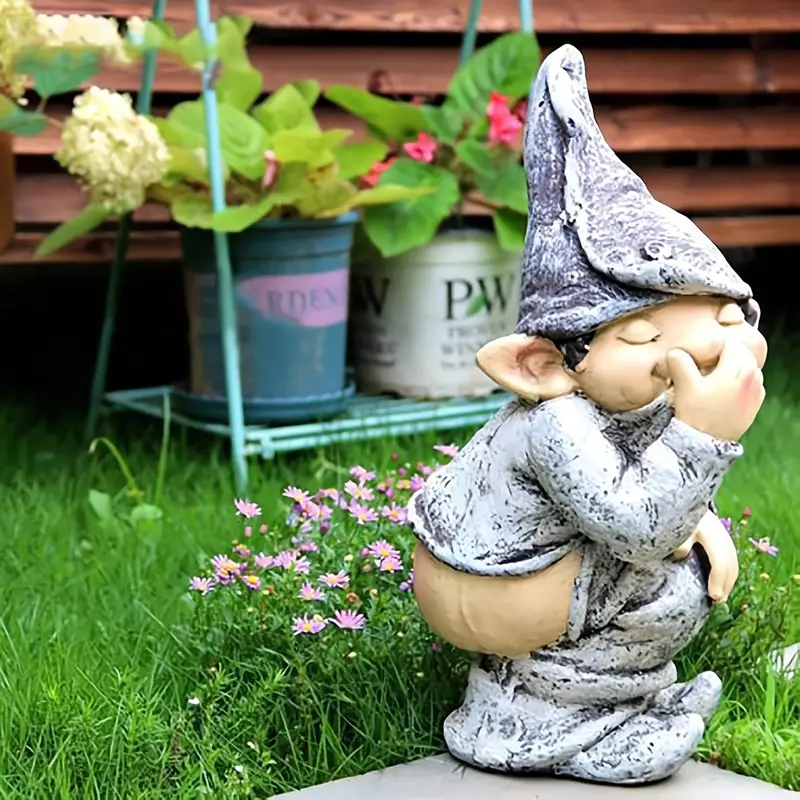In this daytime outdoor scene set in a garden, a whimsical statue of a gnome, with its pants pulled down and nose pinched shut, is squatting humorously on the right side of the image. The gnome appears to be made of concrete and comically looks as if it’s about to relieve himself. Behind it, lush green grass stretches out, dotted with delicate purple asters. To the left, a turquoise metal plant stand holds two potted plants against the backdrop of an old wooden building with lapped wooden siding and brown horizontal wooden beams. The plant on the left sports tiny white flower clusters, while the one on the right is a begonia, vivid with pink blooms. Text reading "PW" is partially visible in the background, adding a touch of curiosity to the charming garden scene.